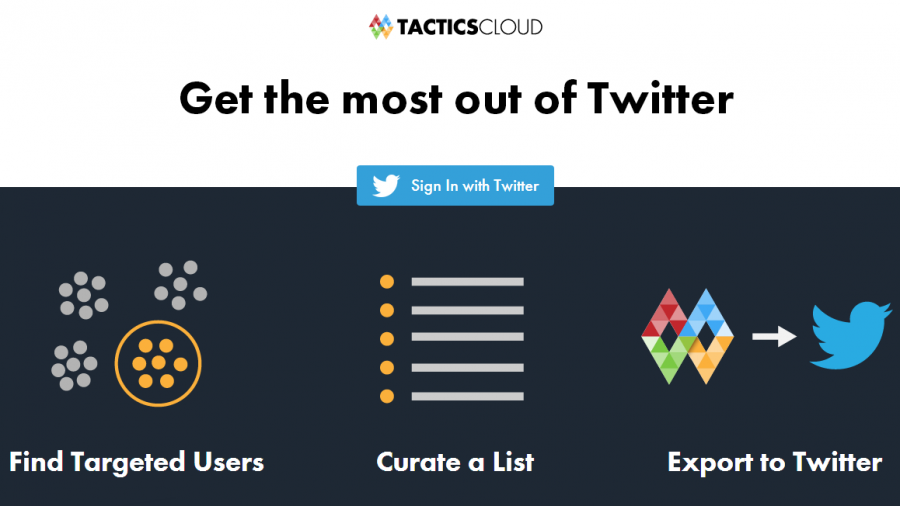The image depicts a webpage designed with a white background occupying the top third and a dark blue background covering the remaining two-thirds. Centered at the top, there is a distinctive diamond shape composed of two triangles: a red one on top and a green one below it. To the right of this diamond, there is another diamond with a blue triangle on top and a yellow triangle on the bottom.

Below these shapes, the text "TACTICS" is prominently displayed in bold black font, followed by "CLOUD" in normal, all-capitalized font. Underneath this title, the slogan "Get the most out of Twitter" is written in bold.

Splitting the white and blue backgrounds is a light blue tab featuring a white Twitter bird icon on the left and the text "Sign in to Twitter" beside it.

On the dark blue background to the left, there is a gray circle surrounded by six smaller gray circles. Further to the right, another gray circle is depicted with five smaller gray circles surrounding it. Below this, there is another gray circle with six smaller gray circles around it, and to the left of this is a yellow-outlined circle filled with a yellow circle and surrounded by six smaller yellow circles.

In the bottom left corner, "Find Targeted Users" is written in bold white text. Centrally located are five vertically aligned yellow dots with horizontal gray lines extending approximately two inches to the right of each dot, spanning all five dots. Below this, "Curate a List" is displayed in white.

Reappearing at the bottom are the same diamond shapes as at the top: one with a red top triangle and green bottom triangle, and another with a blue top triangle and yellow bottom triangle. To the right is a white arrow pointing right, with a blue Twitter icon beneath it. "Export to Twitter" is written in white below this icon.